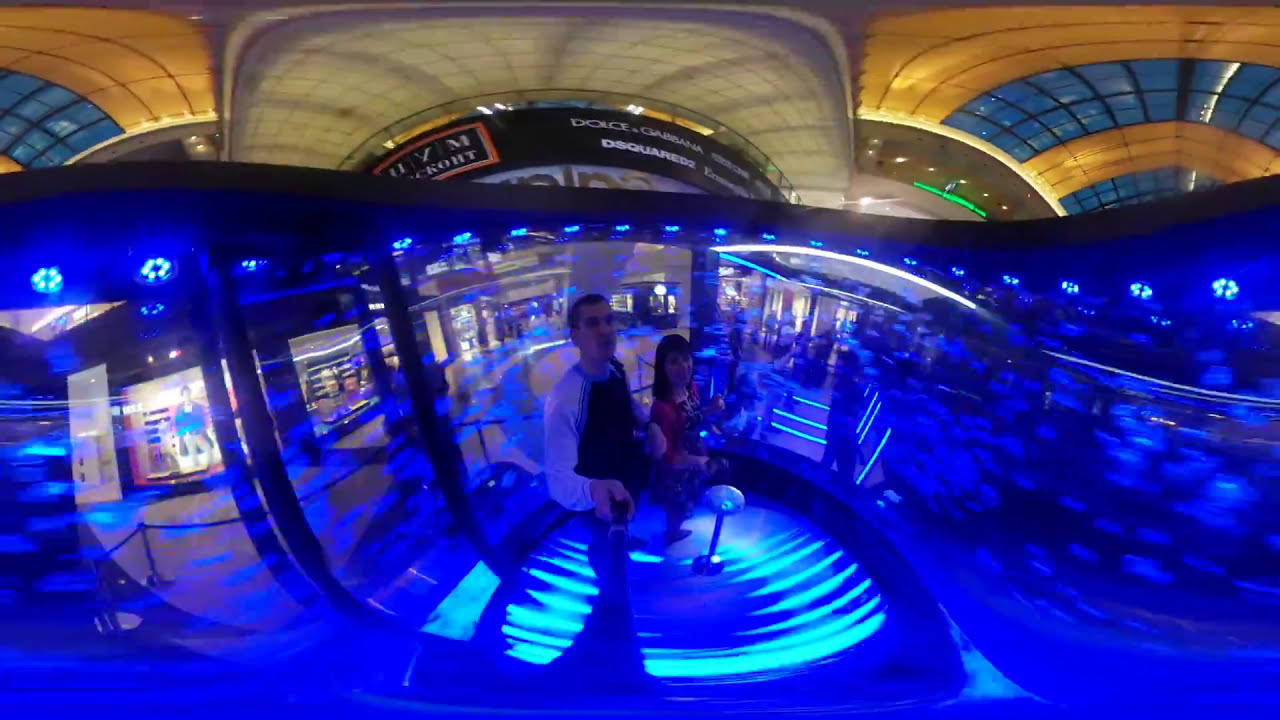The image depicts a peculiar blue-lit area within a mall, which gives off an amalgamated vibe of a nightclub and a science lab. This specific spot might be a photo booth or a karaoke bar, as speculated from the setup. The location is somewhat dark, accentuated by blue lights both above and from the ground, casting an ambient glow. Behind the scene, recognizable stores such as Dolce & Gabbana, D Squared, Adidas, and HYM are visible, confirming the mall setting.

In the foreground, a man dressed in a black-and-white t-shirt with blue borders and shorts is taking a selfie using a selfie stick. The smartphone or camera he is using appears to have a blue filter over the lens, adding to the blue-tinted atmosphere. Standing next to him is a young woman, complementing the odd yet intriguing environment of this mall at dusk, beneath a ceiling adorned with windows.